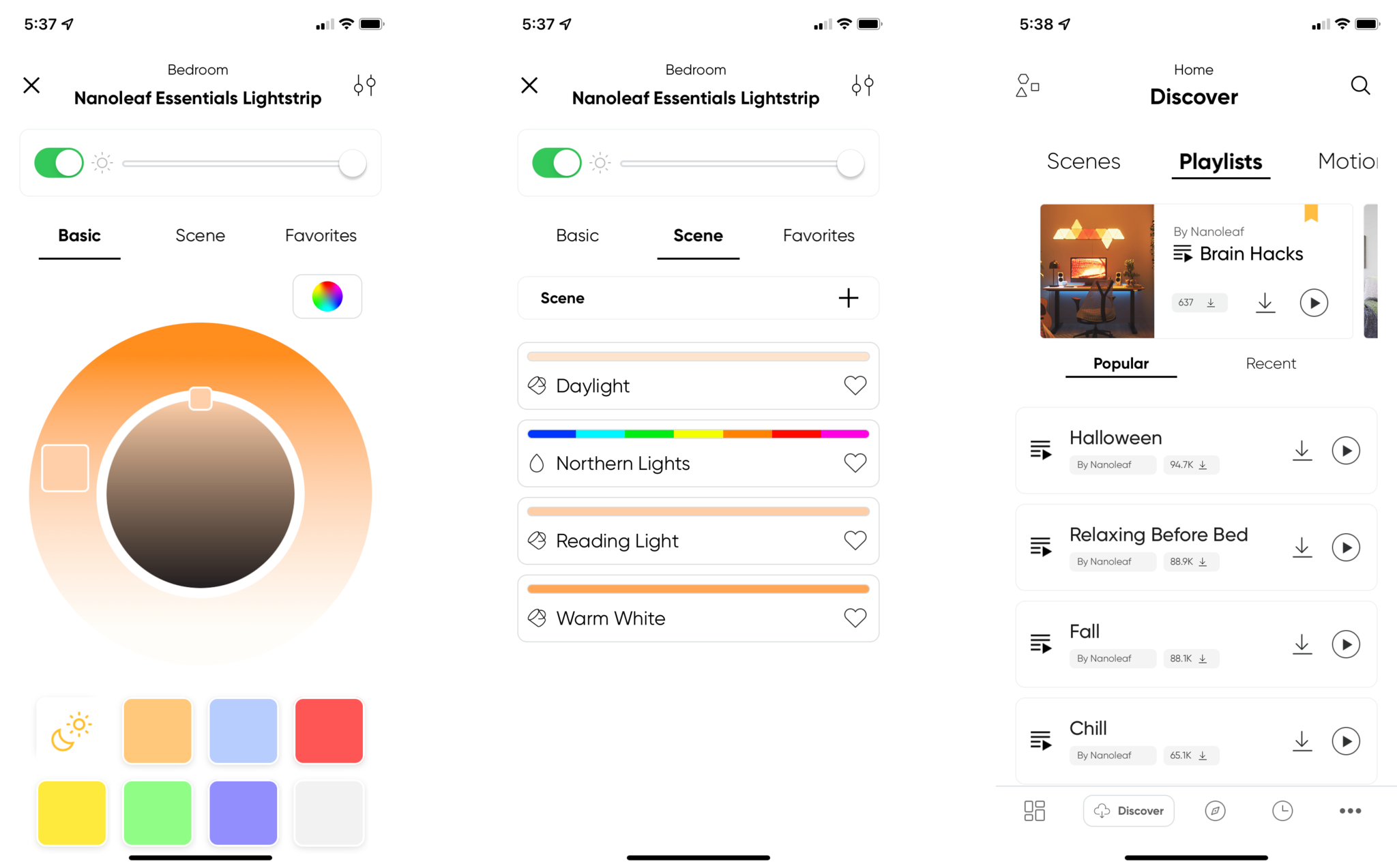This image consists of three side-by-side screenshots, arranged in three columns, illustrating the features of a smart home lighting app.

**Left Column:**
The first screenshot displays the interface at timestamp 5:37 on a cell phone. It shows control options for the "Bedroom" and specifically the "Nanoleaf Essentials Lightstrip." A green toggle indicates that the light is turned on and set to 100% brightness. The interface shows tabs for "Basic," "Scene," and "Favorites." The selected color appears to be an orange hue with a brown center.

**Middle Column:**
In the second screenshot, also at 5:37, the interface shifts to the "Scene" tab, offering several preset lighting scenes including "Daylight," "Northern Lights," "Reading Light," "Warm," and "White." These presets allow the user to quickly change the color and ambiance of the lighting.

**Right Column:**
The third screenshot, now timestamped at 5:38, reveals additional options within the app including playlists. Highlighted is a playlist labeled "Brian Hacks." Additional popular playlists shown include "Halloween," "Relaxing Before Bed," "Fall," and "Chill." This section suggests that the app not only controls lighting but also integrates music to create specific moods and atmospheres in each room.

Overall, the app appears to offer a comprehensive solution for both lighting and music, enabling users to create and control various ambiances in their home seamlessly.